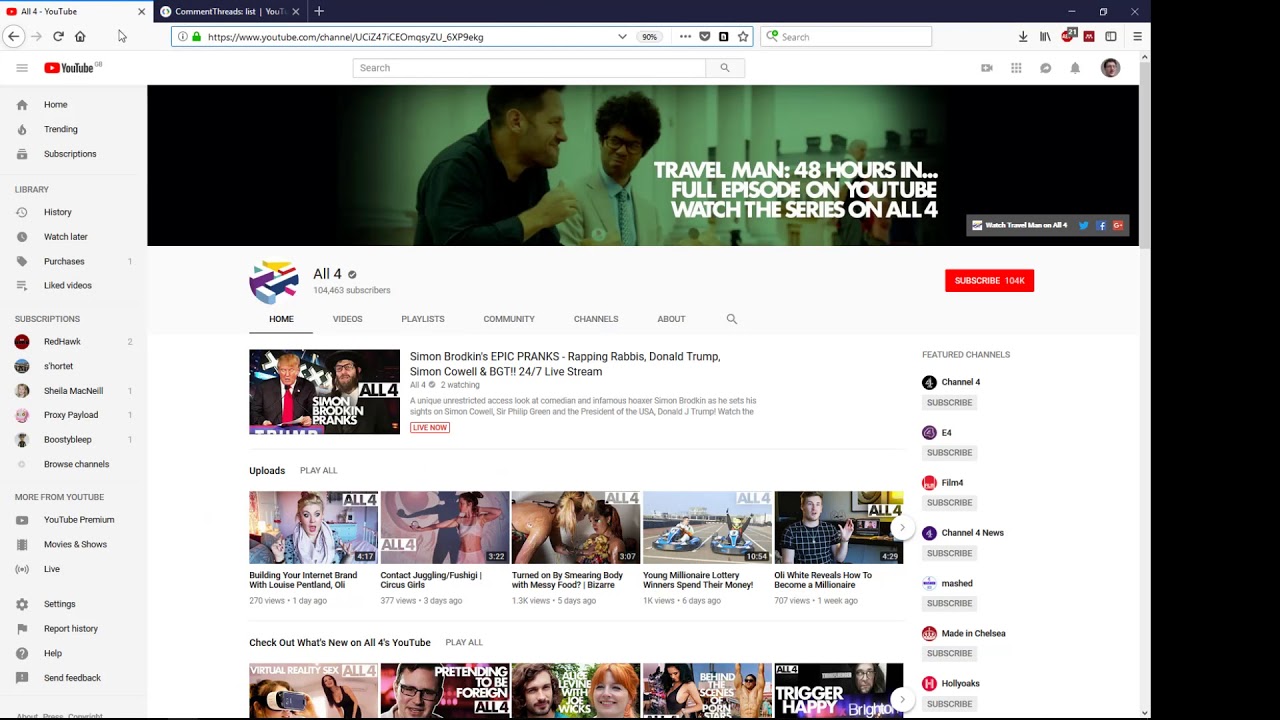The image displays various user interface elements in a colorful and detailed layout. At the top of the image, a blue box is present alongside a small red YouTube icon. To the left, there is a circular icon with a left arrow. A row of icons is positioned nearby, accompanying a large search box, followed by another search box underneath it.

Above these elements, a black box stretches across the top and extends down the right side of the image. Inside this box, the word "YouTube" appears in a white box, situated above another blue box showcasing trending topics and various headings.

To the right side, a white box features a search box along with several icons and a small circular profile picture. Below, there is a contrasting black-bordered image with a greenish background depicting a man and a woman. The caption on this image reads, "Travel Man 48 Hours In, Full Episode on YouTube. Watch the series on All 4." Beneath this image, a small black button is visible.

A light blue box further down contains multicolored blocks in shades of blue, purple, and yellow, labeled "All 4." To the right of this box, a red button is present. The image also includes several tabs and a photograph of Donald Trump engaged in conversation, followed by multiple smaller pictures depicting different shows in a grid format. Beside these, there are names of individuals and small icons aligned to the right.